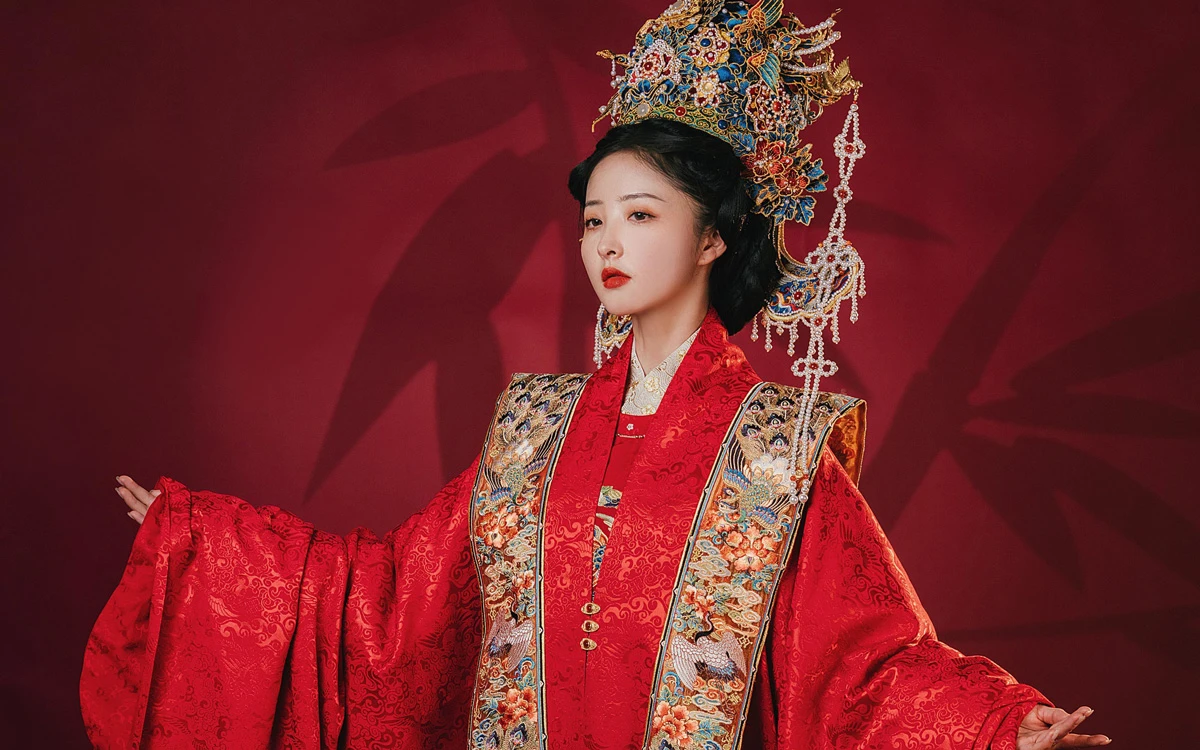The image depicts an Asian woman, likely of Chinese ethnicity, standing indoors and dressed in an elaborate, traditional outfit reminiscent of a Ming Dynasty Chinese wedding dress. She wears a striking, ornate crown decorated with vibrant metal flowers in hues of blue and red and adorned with intricate designs of bird wings and other motifs. The crown features multiple strings of pearls draping down her back. Her face is painted white, complemented by vivid red lipstick.

Her predominantly red, lavish robe features long, flowing sleeves that extend past her hands and resemble wizard sleeves. The outfit includes two sashes on either shoulder, embellished with intricate embroidery of birds, flowers, and other wildlife, predominantly in colors like green, gold, blue, and red. The robe’s front, which has a vest-like appearance, buttons up with three visible buttons and showcases a similar floral and avian motif.

The backdrop behind the woman is a solid red wall, decorated with a silhouette of bamboo leaves, either printed or projected, adding a traditional and serene ambiance to the photograph.